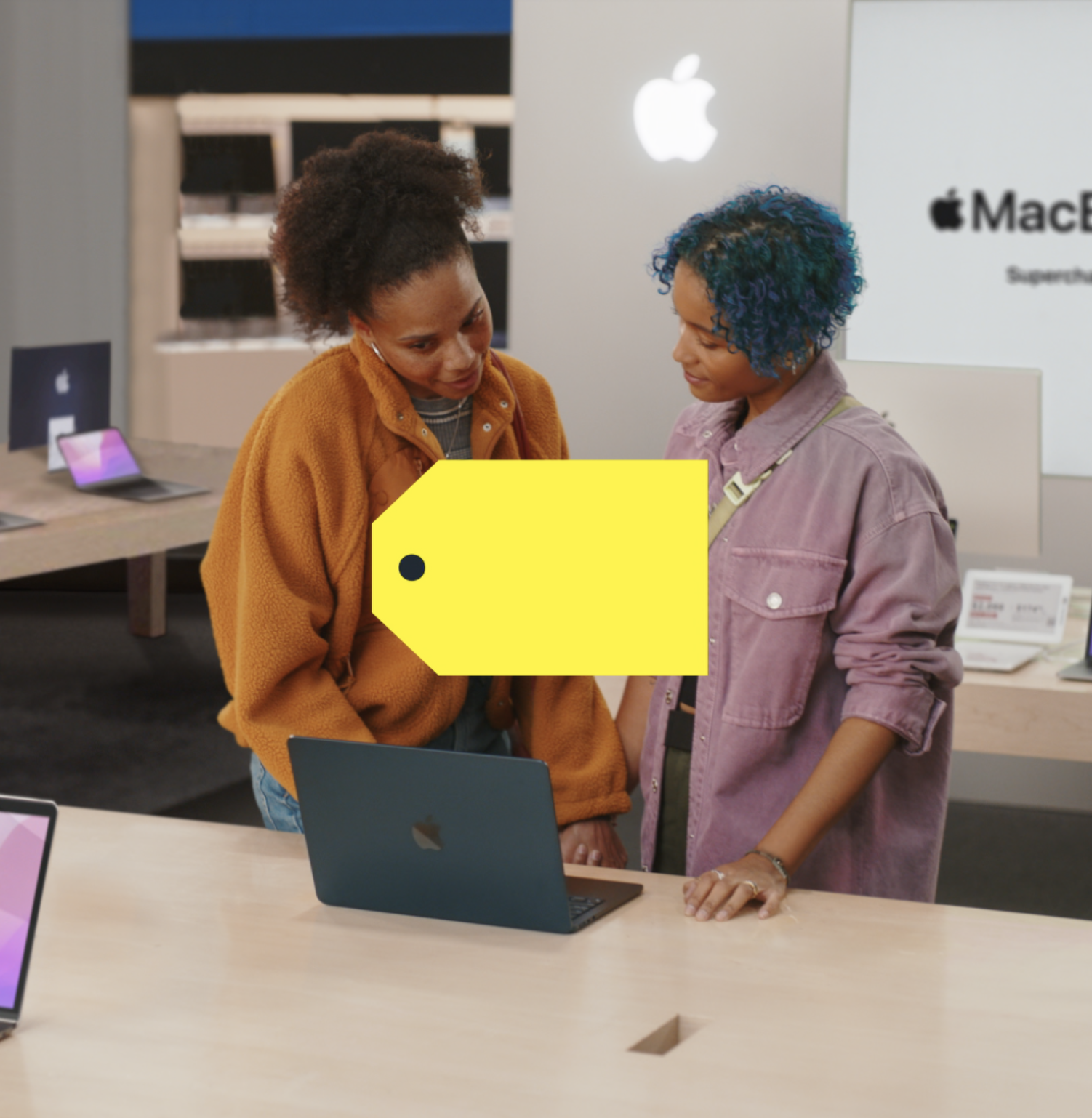This photograph captures an interior scene of an Apple Store, prominently featuring two darker-skinned women interacting with a gunmetal-colored laptop that bears the unmistakable Apple logo. Dominating the center of the image is a large, gold and black price tag that obscures part of the view.

The first woman, with brown curly hair styled in a bun, is attired in a mustard-colored jacket over a gray and white striped shirt. Hoop earrings and a necklace add to her ensemble, which is completed by denim jeans. She is focused on the laptop before her, examining its screen with keen interest.

Standing beside her is another woman with curly, dyed blue hair. She is dressed in an oversized lavender denim jacket with the sleeves stylishly rolled up, revealing a dark shirt underneath. A tan purse strap is visible around her neck area, and she accessorizes with rings on her fingers and a bracelet or watch on her wrist. Her dark pants complement her overall look. She too is engrossed in the laptop, sharing the same focus as her companion.

The laptop they are examining rests on a blonde wood table. Nearby, partially visible, is another black laptop displaying a pinkish-lavender screen. The background is filled with more Apple products, including white and silver laptops on display tables. The back wall clearly displays the word "MacBook" along with the iconic Apple logo in gray. Between the two women's heads, a lit Apple logo glows brightly. Additional laptops and store elements can be seen in the distance, contributing to the bustling ambiance of the store.